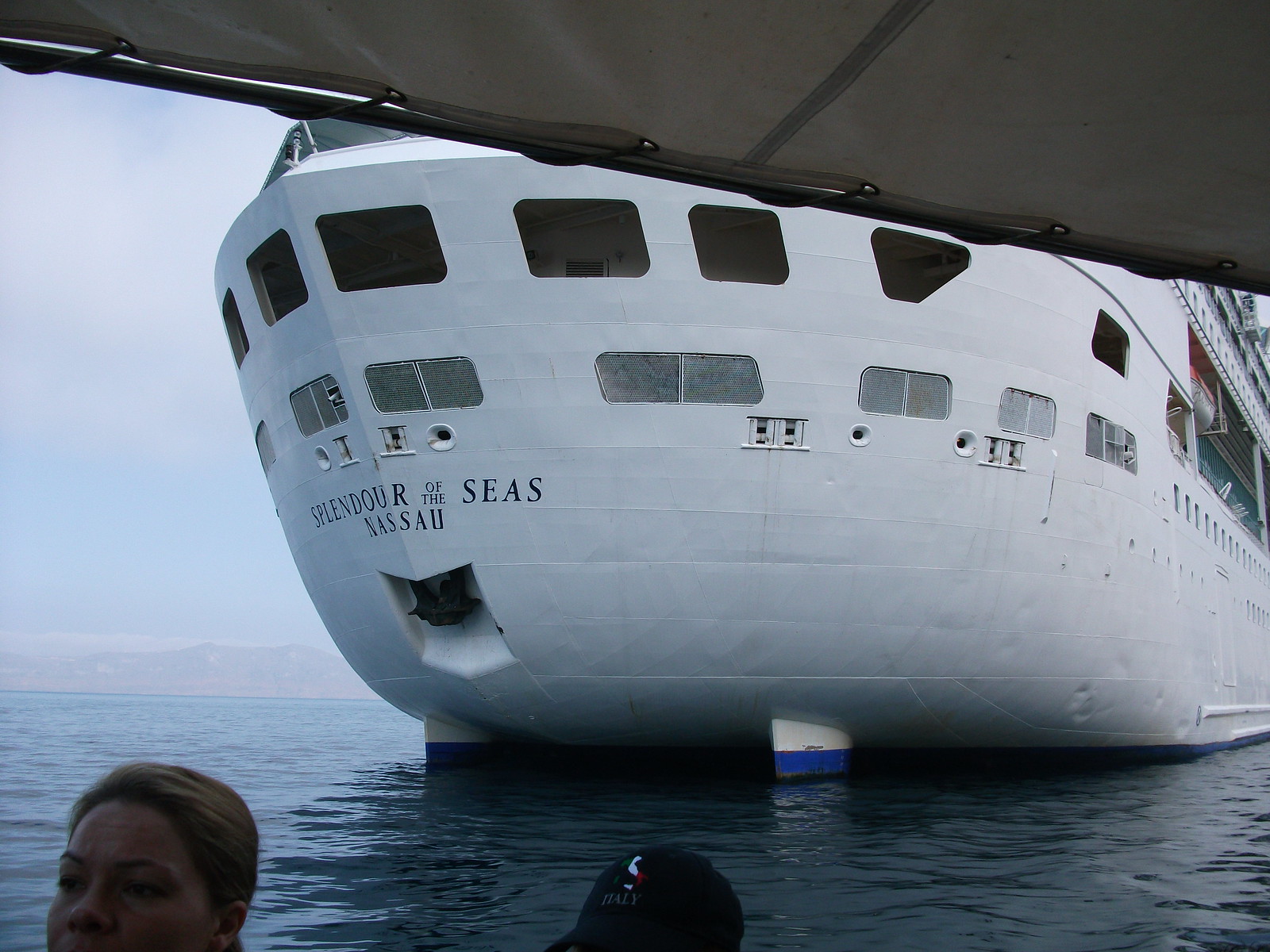The image captures a bright and clear sunny day with a vivid blue sky and a few white clouds. Dominating the scene is the formidable white cruise ship, **Splendor of the Seas, Nassau**, with the name prominently displayed at both the stern and the bow. The vessel features three to four stories, numerous portholes, and wider windows at the stern. Visible alongside the stern are its two rudders, characterized by their white tops and blue bottoms. The ship appears to be docked or anchored on exceptionally clear blue water, with a mountain range forming the picturesque backdrop.

In the lower left corner of the photograph, partially obscured by the framing, are the heads of two individuals. One of them is identifiable as a woman, while the other's gender is indistinct, but this person is wearing a hat emblazoned with the word "Italy." Additionally, a section of what seems to be a sail or canvas overhangs to the upper left and right in the photograph. Notably, the image is devoid of other ships or boats, focusing solely on the majestic cruise liner and its serene environment.